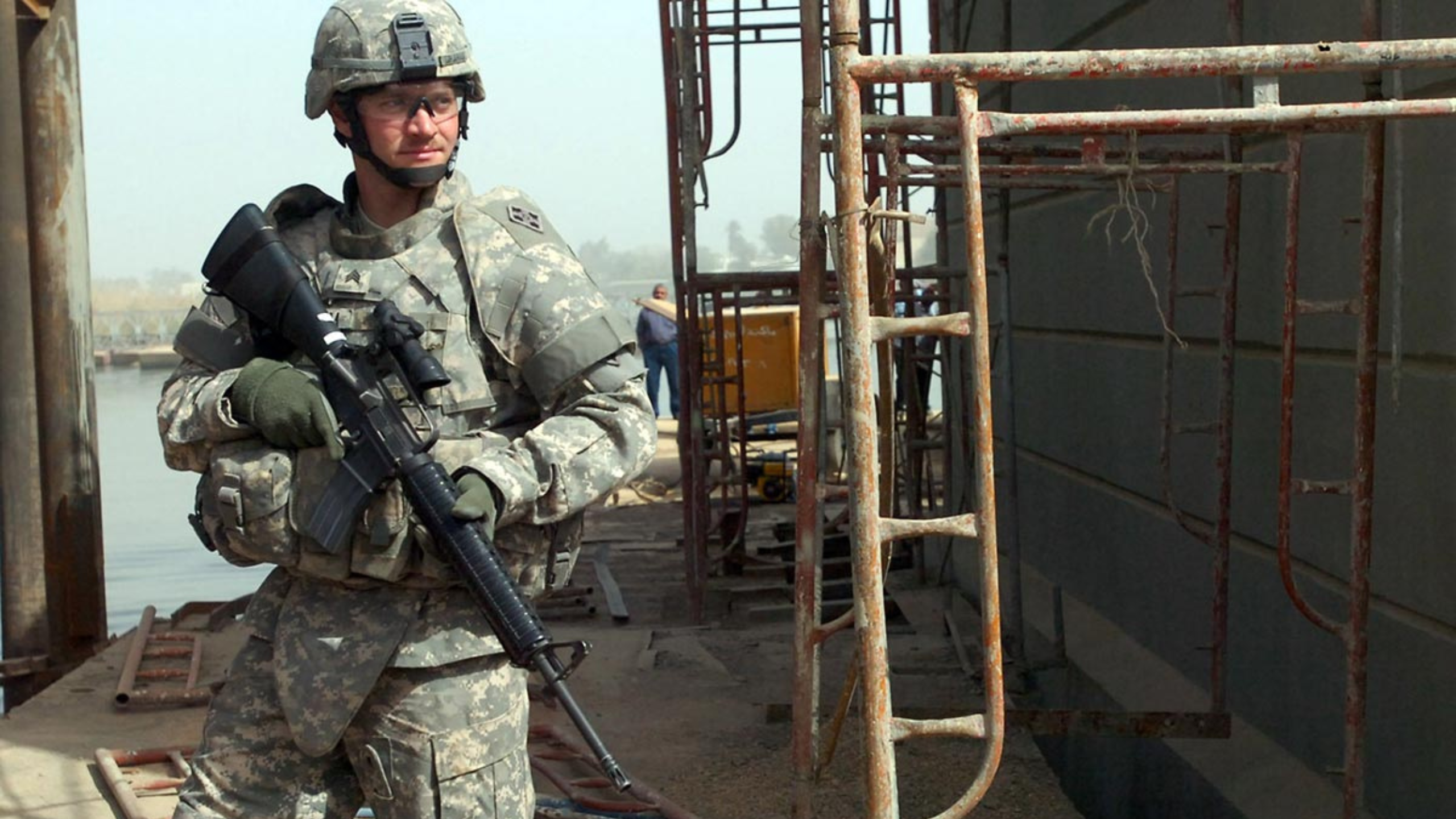In this detailed photograph, a young soldier, dressed in modern U.S. Army gear, stands on guard in an industrial setting. He is attired in gray camouflage with a helmet mounted with a flashlight, protective goggles, and green gloves. The soldier, who appears to be a sergeant with the rank insignia on his chest, holds a semi-automatic rifle, likely an M16, firmly in both hands. The scene behind him reveals a landscape of scaffolding, rusted metal structures, and ladders, suggesting an ongoing construction project. The soldier stands on a cement walkway beside a gray brick building, with another civilian in jeans and a T-shirt visible in the distance. The background shows a water body with a shore dotted with trees and buildings, under a heavily smog-filled sky. This solemn, vigilant figure seems to be tasked with protecting the area, standing alert and facing the camera amidst the industrial chaos.